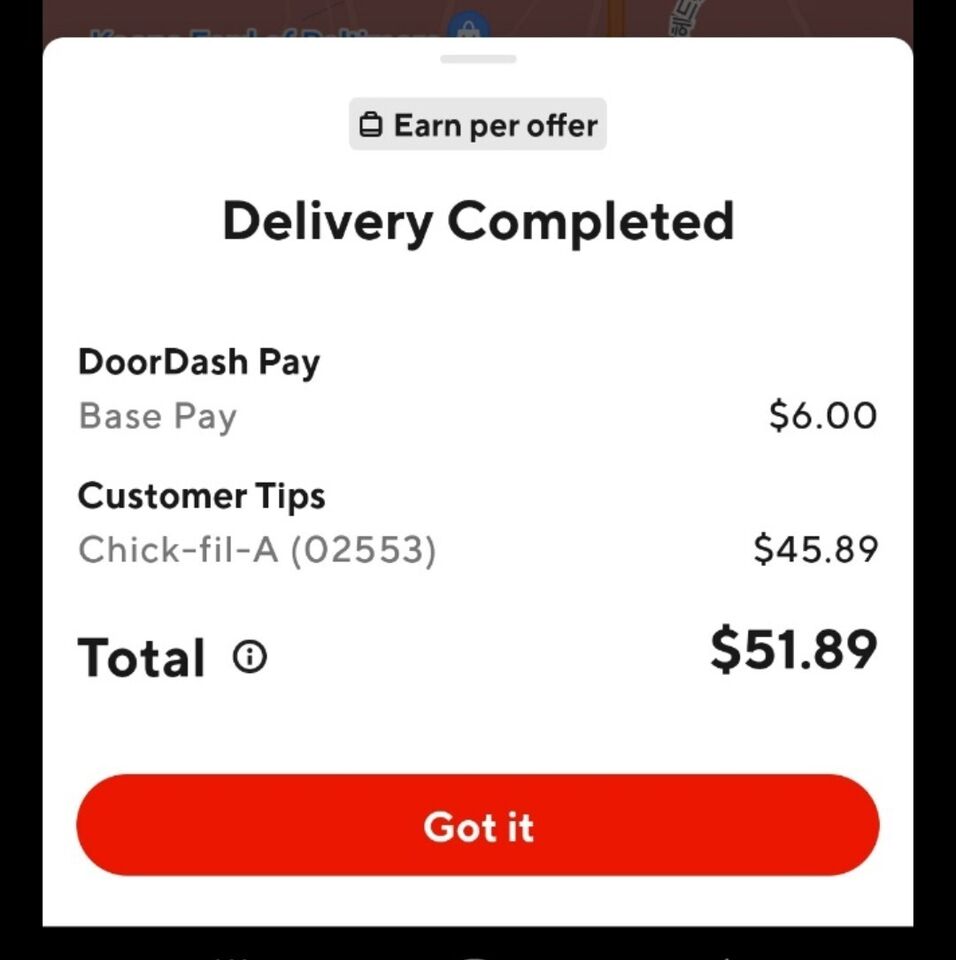The screenshot captures a pop-up message with a black-bordered square overlaying a background that shows a hint of a pink line at the top. The pop-up message itself is primarily white, featuring a gray header centered at the top which reads "Earn per offer." Below the header, the main message in bold text states "Delivery completed." Underneath that, in plain text, it says "DoorDash Pay" followed by "Base Pay" with "$6" displayed to the right. Further down, it mentions "Customer Tips: Chick-fil-A 02553" and "$45.89" to the right. The total earnings shown are "$51.89." At the bottom of the pop-up, there is a large red button that says "Got it" in a small font. The pop-up appears to be a receipt for a DoorDash driver, indicating that they earned $6 for the delivery and received $45.89 in tips, for a total of $51.89. The design could be improved by better utilizing the space on the red "Got it" button for the text.